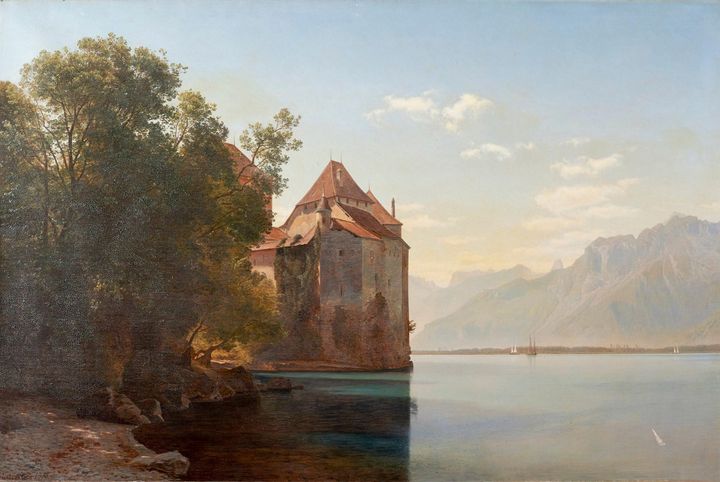This rectangular oil painting depicts a tranquil landscape featuring an ancient historic castle situated at the edge of a serene blue lake. The castle, with its multi-story stone walls towering up to 50 feet, is adorned with small carved-out windows and topped with a distinctive red triangular roof. The setting sun casts the castle’s shadow onto the lake, giving the water a dark blue hue near the structure. The shoreline on the left is lined with tall, green trees while the calm lake extends towards the bottom right. Small boats are visible floating on the lake’s surface. In the backdrop, there is a faint, towering mountain range painted in shades of light green and brown, contrasting with the bluish-gray sky sponged with wispy white clouds. The tranquil and detailed scene encapsulates the serene beauty of the historic lakeside castle and its natural surroundings.